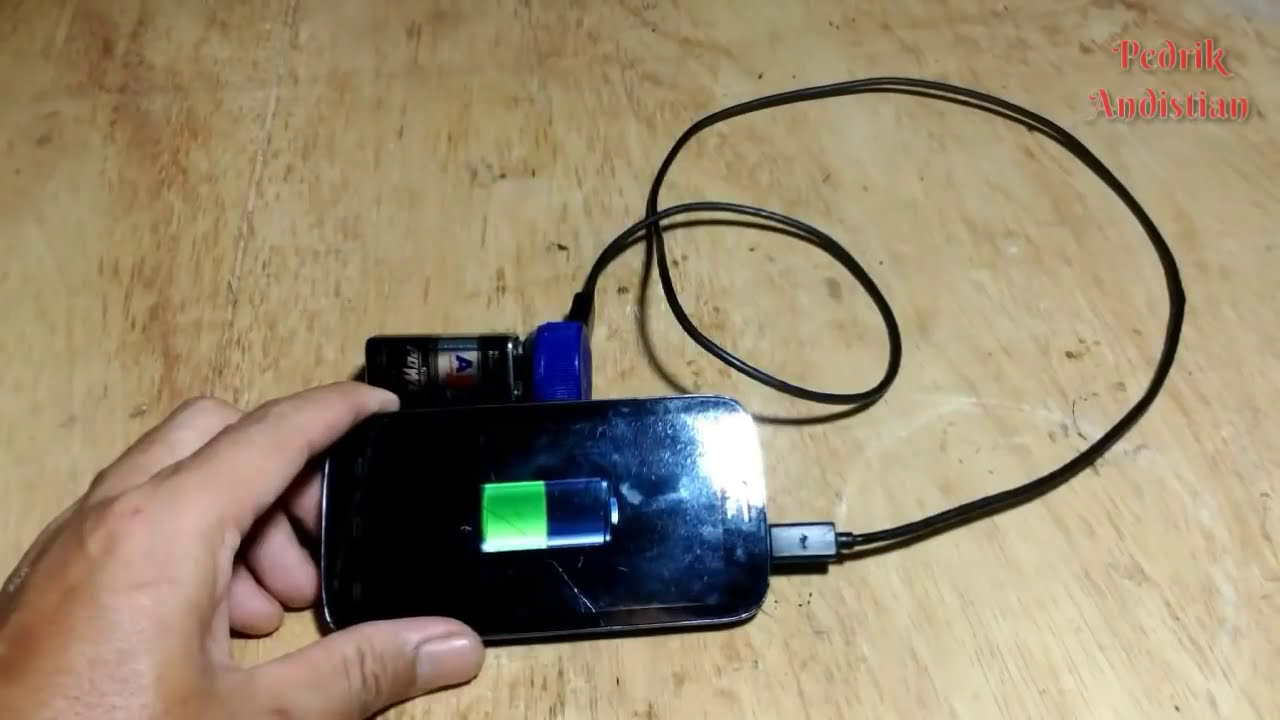A detailed photograph depicts a black cell phone positioned horizontally on a light wooden surface, likely a table or desk. The phone is slightly left of center in the image, with the bottom gripped by a hand that enters from the lower left corner. The hand, which appears to have a tanned or darker complexion, holds the phone between the thumb and index finger, while the other fingers are folded under. The cell phone's screen is black except for a half-full green battery icon, indicating it is charging. A black charger cord is connected to the phone’s bottom right port, looping upward, to the right, then curling back to connect to a portable charger with a blue cap slightly above the phone. In the upper right corner, partially obscured red text appears to say "Pedrick Andisgen" or something similar. The wooden surface, light in color, serves as the backdrop for the entire scene.